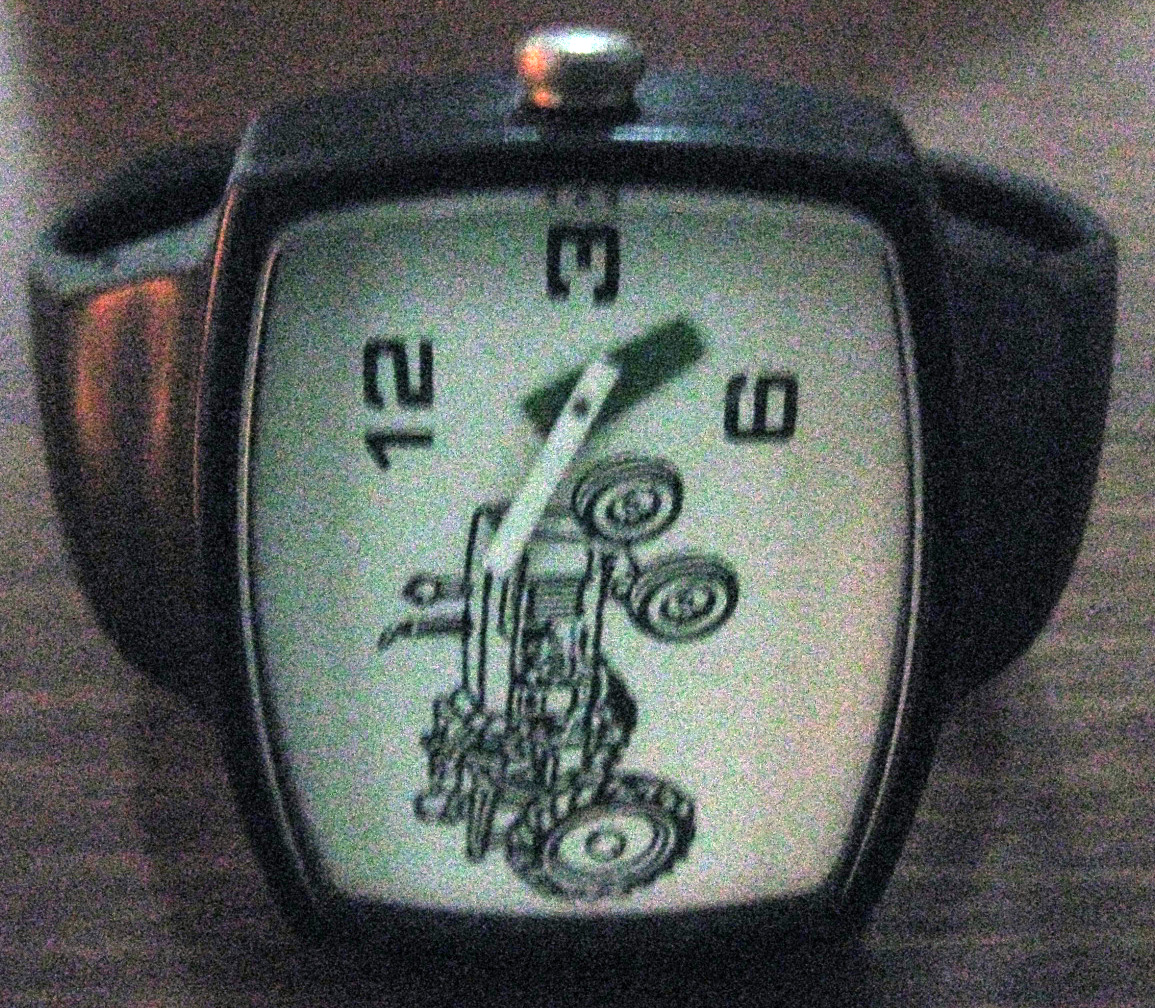This grainy, slightly out-of-focus photo captures a wristwatch lying on its side on a table. The watch features a black band, which could possibly be made of leather or faux leather. The wristwatch has a distinctive square face with a white background. A black illustration of a tractor decorates the face, surrounded by the numbers 12, 3, and 6. The watch's small white hand is also visible against the background, adding to the overall vintage aesthetic of the timepiece.